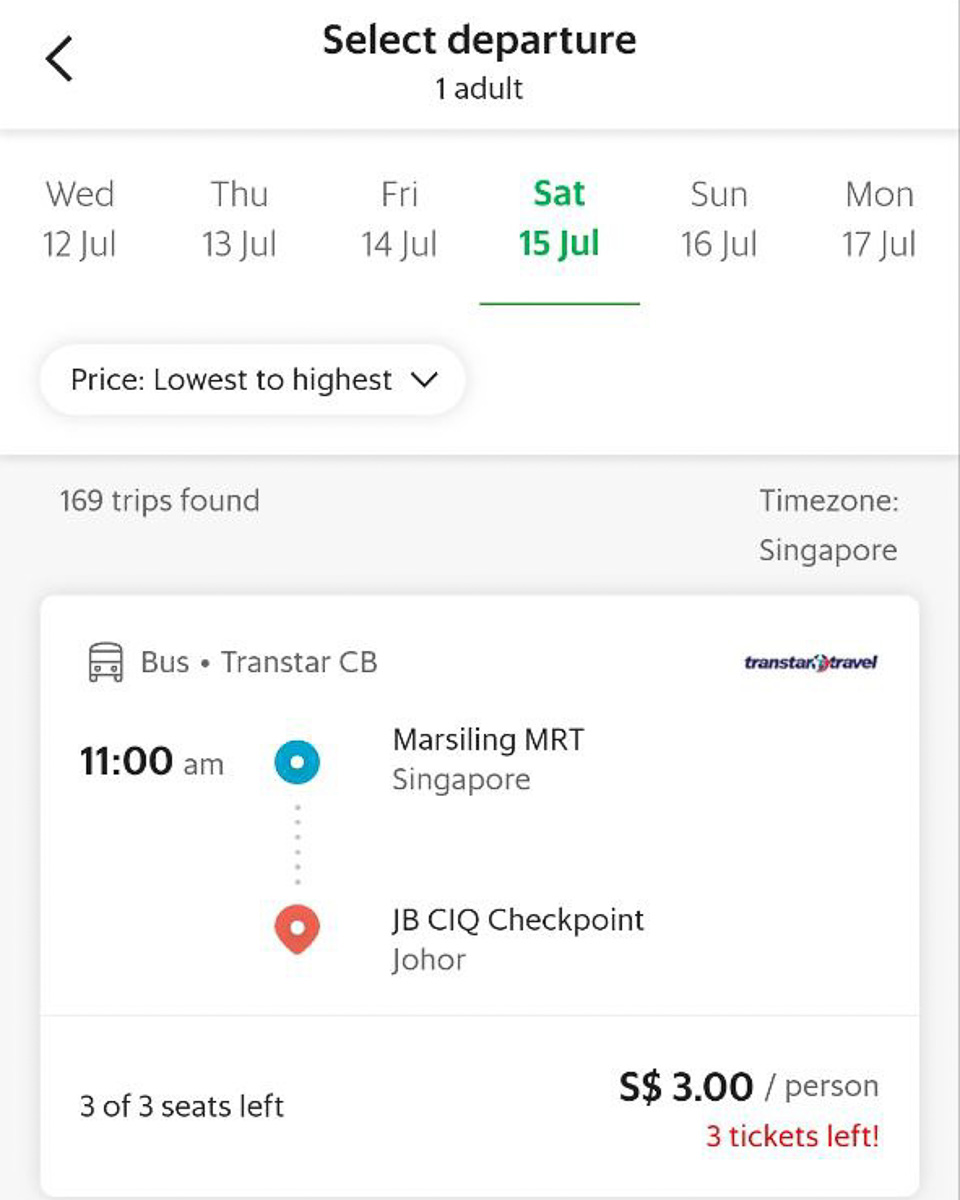Screenshot of a bus station booking website showcasing various options for selecting a bus ticket. In the top left, there is an icon of a left-facing arrow. Centrally positioned, the text reads "Select Departure, One Adult" in black. Directly below, a calendar displays abbreviated days of the week: "WED," "THU," "FRI," "SAT," "SUN," and "MON," corresponding to dates 15th JUL, 16th JUL, and 17th JUL, with the date 15th JUL highlighted in green.

Beneath the calendar, there is a filter option bubble stating "Price, lowest to highest" with a downward-facing arrow. To the bottom left, it indicates "169 trips found". Directly to the right, the text "Time Zone:" appears, followed by the word "Singapore".

Further down, a white box features an icon of a bus with the label "bus" next to it and a small dart symbol. The bus company name "Trans-Star CB" is listed alongside "Trans-Star Travel". Below this, it specifies an 11 AM departure from "Marsiling MRT Singapore", with a red marker indicating the arrival point at "JBCIQ Checkpoint Johor". It notes "3 of 3 seats left" on the bottom left and displays the price as "S$3/person". On the bottom right, the text "3 tickets left" is highlighted in red.